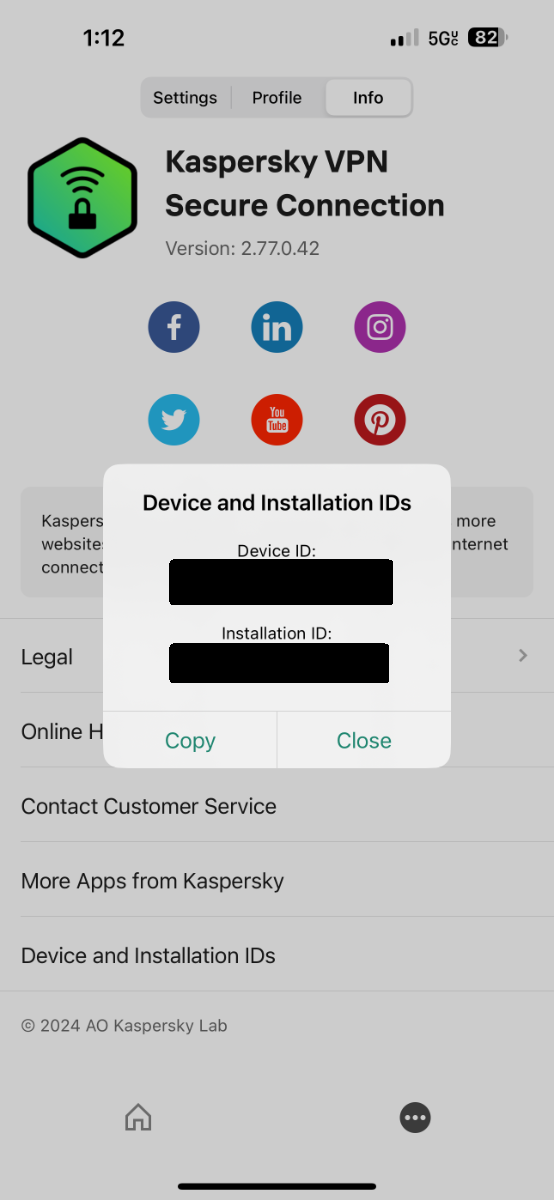In the top left corner of the screen, the time is displayed as 1:12 PM. To the right, a signal icon indicates only two bars of service out of four, represented in black. Adjacent to this icon, a 5G symbol is accompanied by the letters "U" and "C" at the bottom. Further right, a battery icon reads "82," signifying the device is 82% charged.

Below these icons, there's a light gray, oval-shaped menu with "Settings" written in black lettering. A light gray divider separates "Settings" from other options labeled "Profile" and "Info." The "Info" section is highlighted with a white background. Underneath, in black text, it reads "Caspary VPN secure connection," followed by "version: 2.77.0.42" in gray. To the left of this text, an octagon icon features an ombre background of dark and light green, with a black padlock symbol emitting WiFi signals. 

Social media icons for Facebook, LinkedIn, Instagram, Twitter, YouTube, and Pinterest are displayed as circular icons. Below them, a pop-up notification in bold black lettering says "Device and installation IDs," and underneath in smaller black font, "Device ID" and "Installation ID" are both blacked out with long black rectangles. 

At the bottom left of this notification, a "Copy" option is highlighted in blue font, bordered by a light gray area. On the right, a similar "Close" option can be found. Behind this pop-up, a menu is partially visible, listing options such as "legal online help," "contact customer service," "more apps from Caspary," and "device and installation IDs." At the very bottom, the screen features a copyright statement: © 2024 AO Casper sky Lab.

Additionally, a home icon and a dark gray circular icon with three dots—potentially indicating a menu option—are visible at the bottom. The background features a long gray area with black writing, partially displaying the words "Casper's website," "connect more," and "internet."